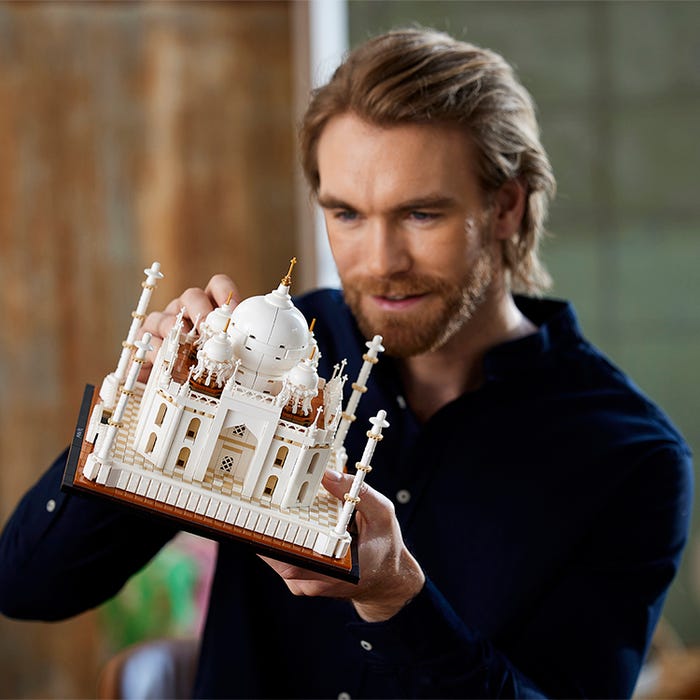The image depicts a man with golden brown hair and a full beard, dressed in a dark blue, long-sleeved button-up shirt. He is holding a detailed model of a white domed building, which appears to be a Lego-like brick-built representation of either the Taj Mahal or a church. This intricately designed model features a large central dome surrounded by several smaller domes and long pillars at each corner adorned with gold rings. The structure is predominantly white with tan windows and sits on a checkered white and tan base. The setting behind the man is out of focus, with hints of tan, green, and pink, ensuring the focus remains on him and the architectural model he is examining.